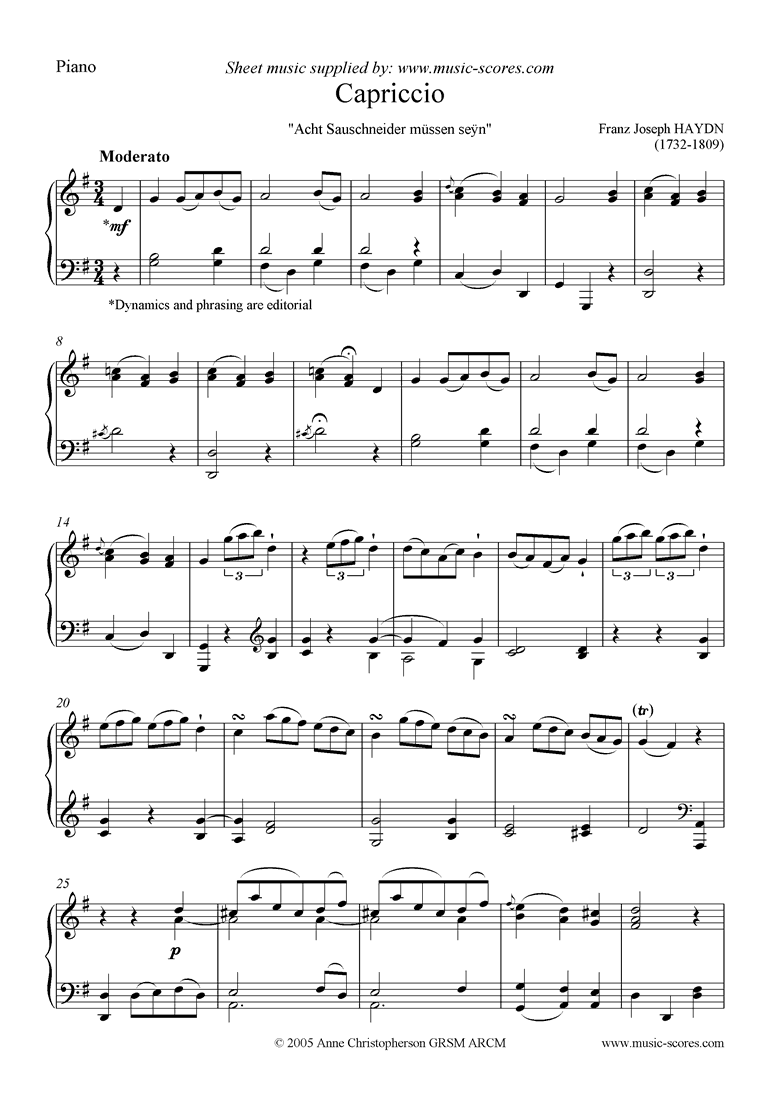The image depicts a detailed sheet music of the piece "Capriccio" specifically arranged for piano, as noted by the word "Piano" in the upper left corner. The sheet music is supplied by www.music-scores.com, and this is printed above the title. Below "Capriccio," there is a German phrase "Acht Sachsehlemmer Museum," followed by the name of the composer, Joseph Franz Hayden (1732 to 1809), indicating it is a historical composition. "Moderato" is marked at the top left of the sheet, guiding the tempo of the piece. The dynamic marking "MF" with an asterisk notes that dynamics and phrasing are editorial. The score consists of ten lines of musical notation, with various clef signs and musical notes including four-note bars and bars of three notes. There are also arches over some notes, and lines are occasionally above or below the notes. The numbers 8, 14, 20, and 25 are positioned above rows, suggesting measures or key points in the score. The bottom of the sheet lists the copyright information as "2005 Ann Christopherson ARCM," with a repeat mention of the source, www.music-scores.com, on the bottom right.